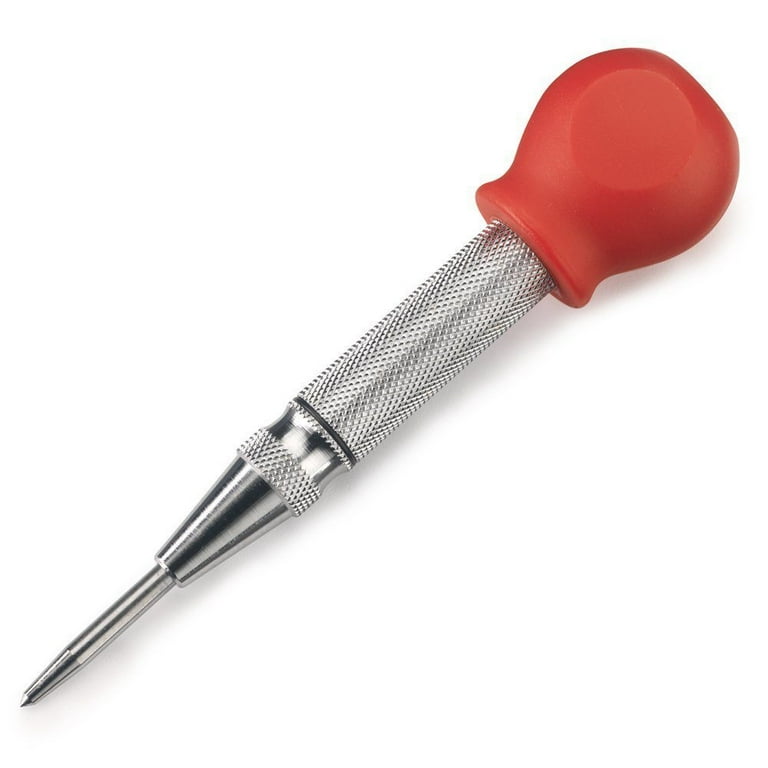The image is a clear, well-lit, close-up photograph of a single silver automatic center punch, placed diagonally from the top right to the bottom left against a bright white background. This metallic tool features a sharply pointed tip at one end and a rounded, red rubber knob at the other end, which is designed for palm pressure usage. The center of the tool showcases some dot-like embossing, and a subtle shadow is cast towards the right side of the object. There are no other items, letters, or numbers in the image.